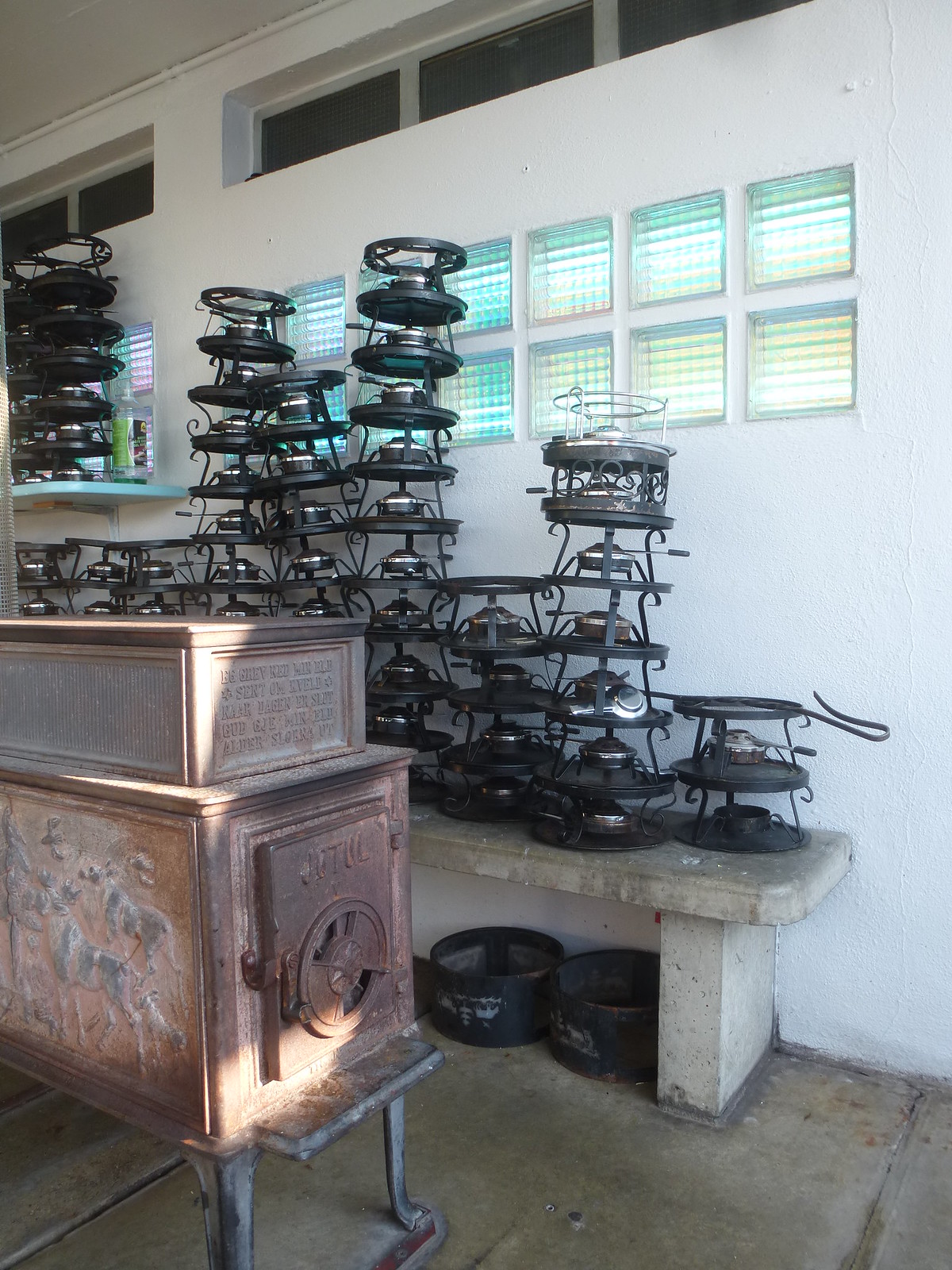The indoor color photograph showcases an organized arrangement of buffet heaters. These circular, black metal heaters, each featuring a silver center burner, are neatly stacked in columns on a stone shelf in the background. The background wall is white and prominently features glass blocks extending from right to left about two-thirds of the way up, which have a blue and green tint, allowing a bit of light to pass through.

In the left foreground, a rugged stone or brick oven extends into the frame, shown in a three-quarters view. The oven's front displays a rectangular door with a circular, adjustable vent. The floor underneath all this appears to be concrete, lending an industrial feel to the scene. Notably, an additional element mentioned is a wooden box with carvings of moose and a circular latch, which stands out against the rest of the metallic and stone textures, though it is not the primary focus of the image. The overall setting is devoid of any text or print, emphasizing the detailed visual elements present.